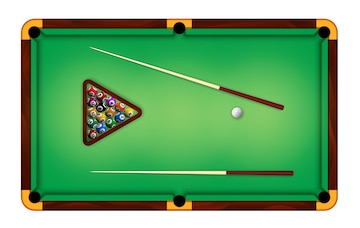This image depicts an animated aerial view of a small replica pool table with a green base and yellow bumpers on the sides. The brown-rimmed table features two pool cues, which are brown at the ends and white towards the tips, positioned with a white cue ball lying between them on the right side of the table. On the left side of the table rests a tilted wooden triangle rack, containing a perfectly arranged set of pool balls. At the top tip of the triangle is a red ball, followed by a purple ball, another red ball, a mustard yellow ball, a black ball, another purple ball, a green ball, a yellow ball, a gold ball, an orange ball, a maroon ball, a bright blue ball, another green ball, a royal blue ball, and another yellow ball, sequentially arrayed downward.